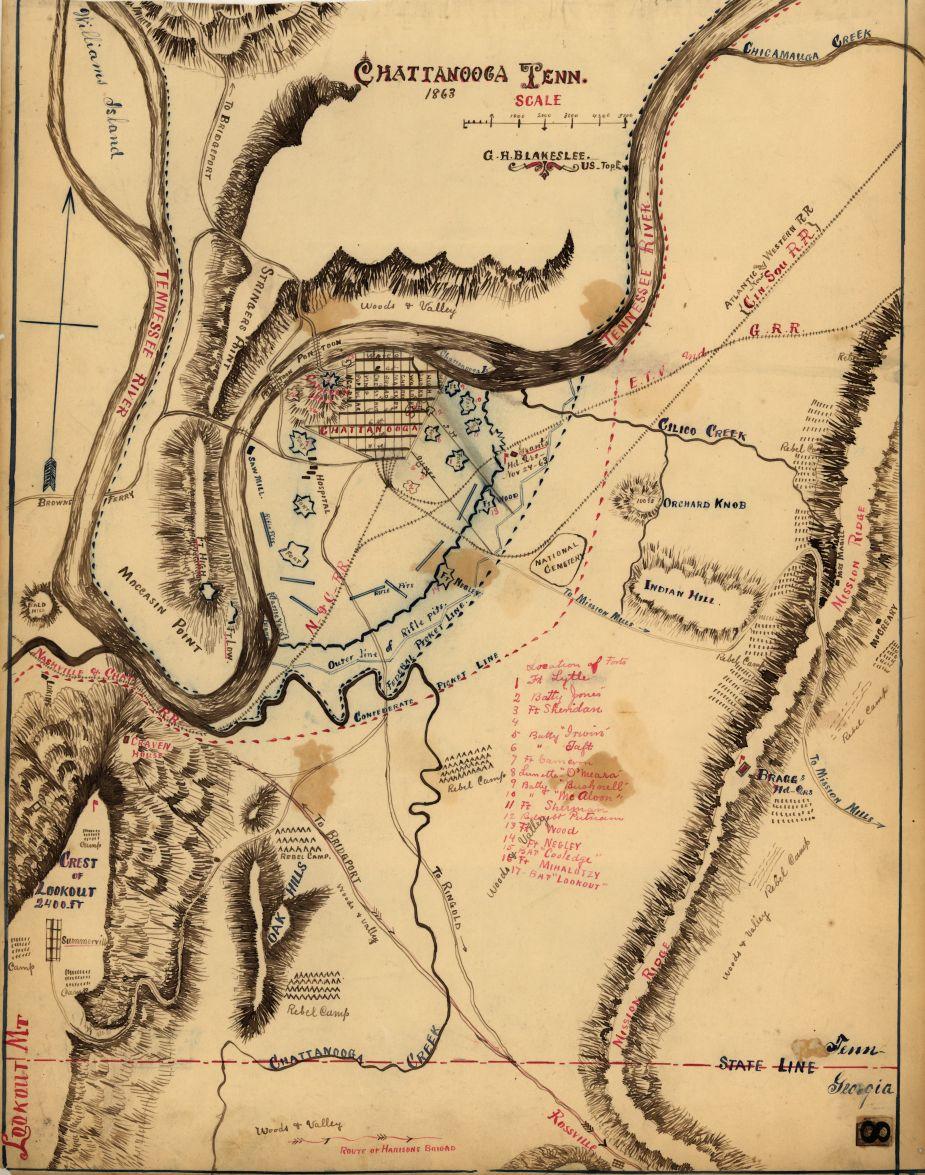This detailed map, reminiscent of those found in fantasy books, is a vintage piece likely from 1863 or 1868, with a header reading "Chattanooga 10" and a title specifying "Chattanooga, Tennessee." The map, which features a cream-colored background with brownish, black, and red inks, portrays a variety of topographical elements including mountain ranges, rivers, and forests. Handwritten notes accompany printed details throughout the map. On the upper left, there's a compass symbol, and beneath the title, a detailed scale measurement is provided. Notable geographic labels include Tennessee River, Chattanooga Creek, Lookout Mountain, Moccasin Point, Williams Island, and Mission Ridge. The map also highlights features such as the Confederate Picnic Line and Rebel Camp, along with various railroads like the Atlantic Western RR, Seamstowe RR, and GRR. Furthermore, significant landmarks like Indian Hill and the crest of Lookout Alt at 2400 feet are denoted. Red ink marks specific divisions and a handwritten list occupies parts of the map, illustrating the thorough and historical nature of this intricate depiction of Chattanooga and its surrounding areas.